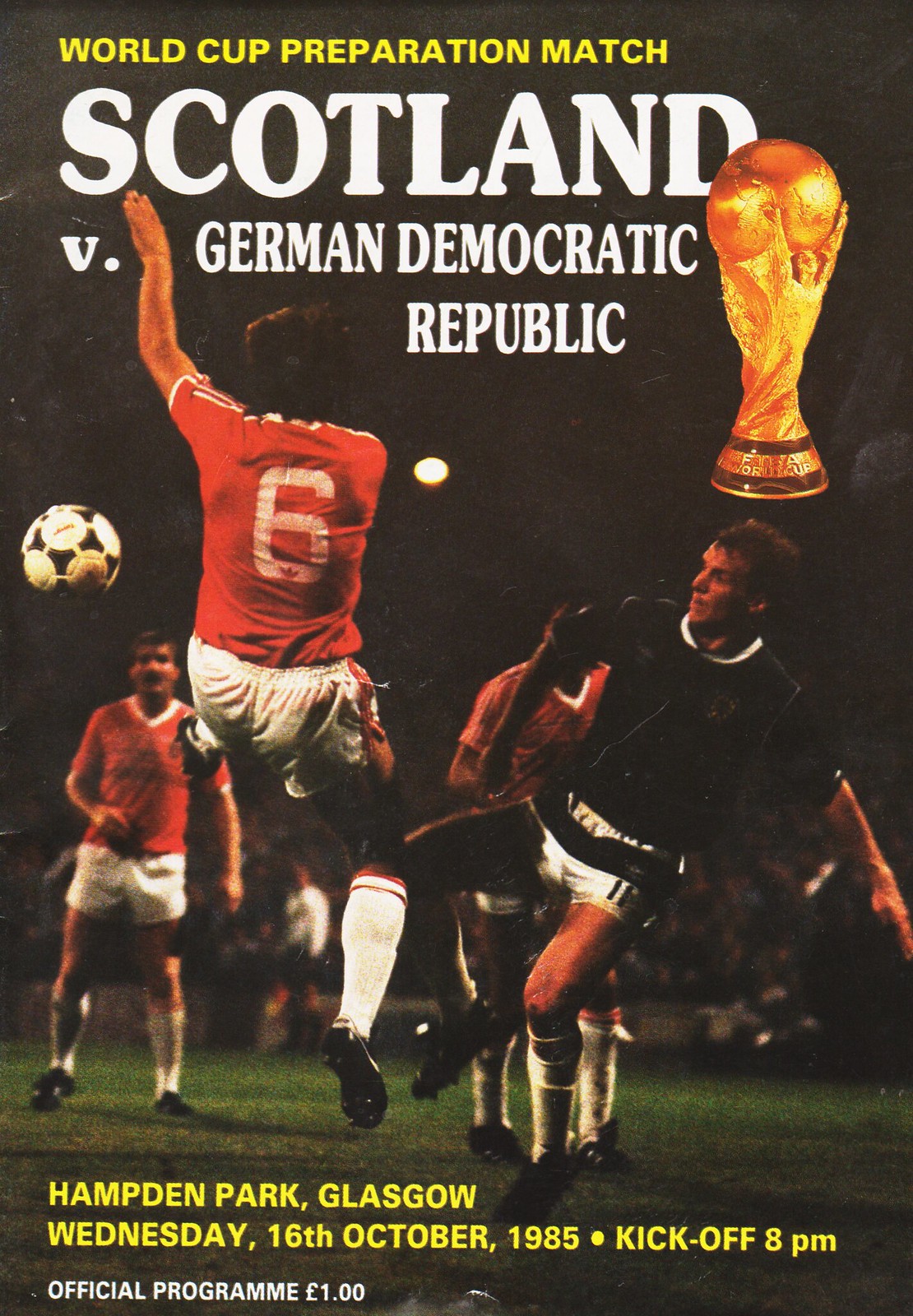The image is a color cover of a vintage soccer program with a black background that gives it a classic, aged appearance with slight browning. It features an action shot from a game between two soccer teams, with one team in red jerseys and white pants and the other in black jerseys and white pants. Prominently, a player in mid-air with a red jersey appears poised to kick the ball overhead, while a player in a black jersey pursues. The ball is visible, soaring through the air. The background shows an audience in the stands, suggesting the match is being played at night, as the lighting highlights the foreground players while maintaining a dark backdrop. 

At the top of the cover, in bold gold letters, it reads "World Cup Preparation Match," with "Scotland versus German Democratic Republic" in white letters below it. Accompanying this text on the top right is a gold trophy resembling a globe held up by angels. Lower down, in yellow letters, the details "Hampden Park, Glasgow, Wednesday 16th October 1985, Kickoff at 8 p.m." are displayed, and the note "official program one British pound" confirms its authenticity as an event program.